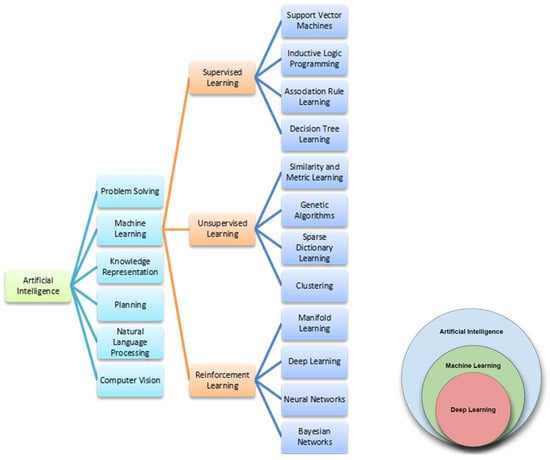This color drawing serves as a detailed overview of artificial intelligence, incorporating both a Venn diagram and a tree diagram to illustrate different approaches and methodologies. On the right, a Venn diagram consisting of three nested circles simplifies the relationships: the largest blue circle labeled "Artificial Intelligence," contains a green circle labeled "Machine Learning," which further contains a smaller pink circle labeled "Deep Learning."

To the left, a comprehensive tree diagram breaks down the facets of artificial intelligence. The root node, labeled "Artificial Intelligence" in yellow, branches out to several key fields in blue boxes: Problem Solving, Machine Learning, Knowledge Representation, Planning, Natural Language Processing, and Computer Vision. Each concept is color-coded for clarity, with green used for specific subfields.

The Machine Learning branch further subdivides into three main types: Supervised Learning, Unsupervised Learning, and Reinforcement Learning. Each of these categories has additional branches detailing specific techniques:

- **Supervised Learning:** Support Vector Machines, Inductive Logic Programming, Association Rule Learning, and Decision Tree Learning.
- **Unsupervised Learning:** Similarity and Metric Learning, Genetic Algorithms, Sparse Dictionary Learning, Clustering.
- **Reinforcement Learning:** Manifold Learning, Deep Learning, Neural Networks, Bayesian Networks.

This meticulous diagram visually organizes and connects AI concepts, demonstrating the hierarchical and interrelated nature of artificial intelligence, machine learning, and deep learning.